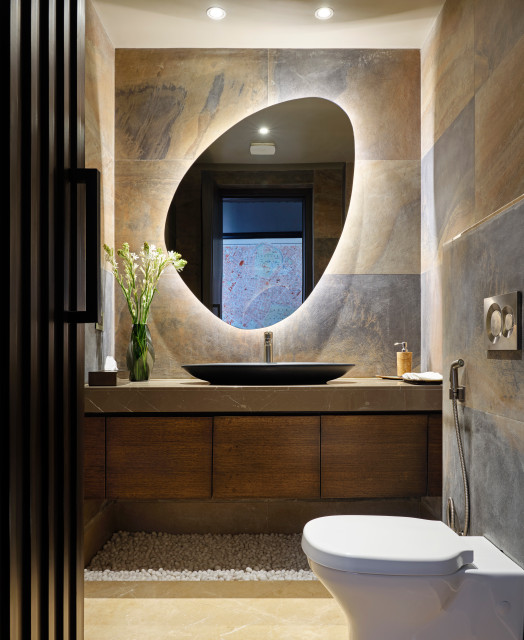This image depicts a very modern bathroom photographed indoors. The shot is rectangular, measuring approximately five inches high by three inches wide. The bathroom features a sophisticated design accented by a blend of natural elements and sleek surfaces. On the right, a wall made from large sheets of brown and gray rectangular stone forms the backdrop. Against this wall stands a tankless, one-piece white toilet, which appears to have a bidet attachment. Just behind the toilet, a silver water sprayer is visible, adding functionality to the space.

The countertop in the background is brown and complemented by brown wooden drawers below. Decorative white pebbles or river rocks are neatly placed at the bottom, suggesting an earthy, Zen-like aesthetic. The sink, positioned on the countertop, is an elegant shallow gray bowl with a single faucet. To the left of the sink stands a green vase holding white flowers, adding a touch of nature and brightness to the room. A soap dispenser is also present on the countertop, enhancing the usability of the area.

Above the sink, an egg-shaped mirror hangs on the stone wall, titled with its narrower end pointing to the upper right. The area surrounding the mirror is bordered with white marble, creating a striking visual contrast. The ceiling of the bathroom is light tan and features recessed lighting that softly illuminates the space.

On the left side of the photograph, a dark brown folding door slides open, revealing a large rectangular handle at its vertical center. The modern design of the bathroom is further emphasized by a plush white rug on the cream-colored floor, providing both comfort and style.